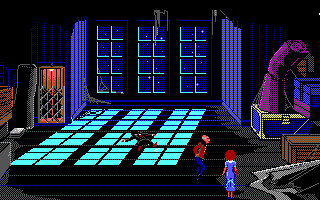In this rectangular image, we find ourselves immersed in a digital game scene depicting the eerie interior of a dilapidated building at night. The atmosphere is unsettling as we observe the large room illuminated by moonlight streaming through three tall windows that span from floor to ceiling. The windows cast stark shadows across the floor, adding to the ominous setting. 

On the floor, there is a figure lying seemingly dead or immobile, positioned towards the center of the scene. To the lower right of the room stands a man and a woman, facing each other. The woman, with her back to the viewer, has brown hair and is dressed in a blue dress. The man, opposite her, is wearing blue pants and a brown long-sleeve shirt.

Adjacent to the pair, also in the lower right corner, is a collection of chests filled with items. There is a brown chest on the floor, above that is a blue chest, and perched on top is a chest painted in shades of blue and purple.

On the left side of the image, a gated metal door adds to the building's fortified appearance. Nearby, a stack of black tires lends an industrial feel to the space. The penetrating light from the high windows throws elongated shadows across the scene, intensifying the sense of foreboding that permeates the game setting.